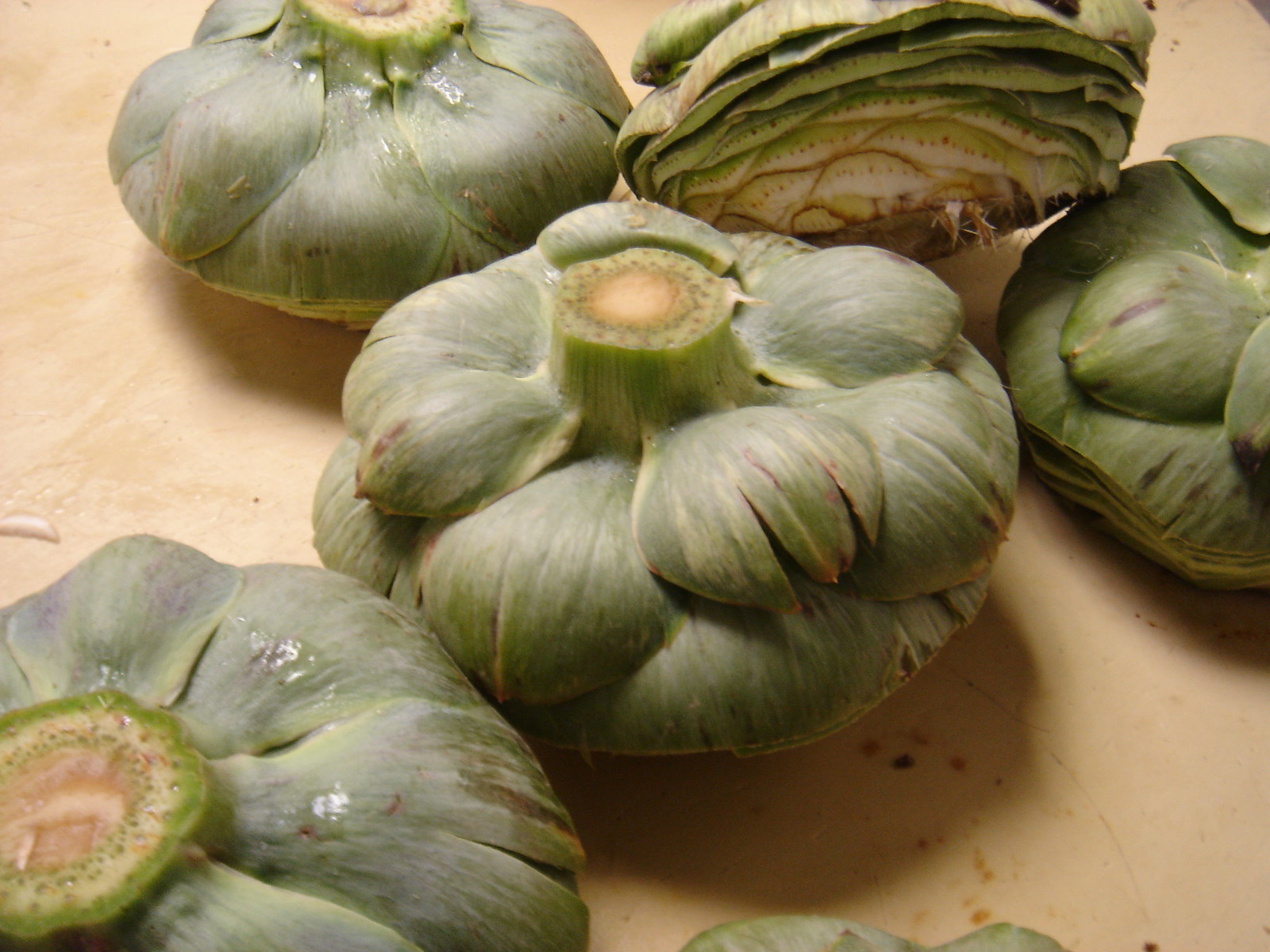The image depicts several artichokes resting on a slightly dirty brown cutting board with a creamish-brown hue, resembling plywood. Most of the artichokes are standing upright with their stems pointing upward, while one has been sliced to reveal its interior. The artichokes display a range of colors, including yellow stems, green leafy exteriors, and areas of brown with light brown dots, and dark green rims. The cut artichoke reveals layered leaves in shades of white, yellow, and light green. The artichokes appear weathered and slightly slimy, suggesting they have been recently purchased and are unwashed. The setting seems to be a kitchen, possibly in preparation for dinner or making a dip. The photograph captures a well-lit scene in a square frame.